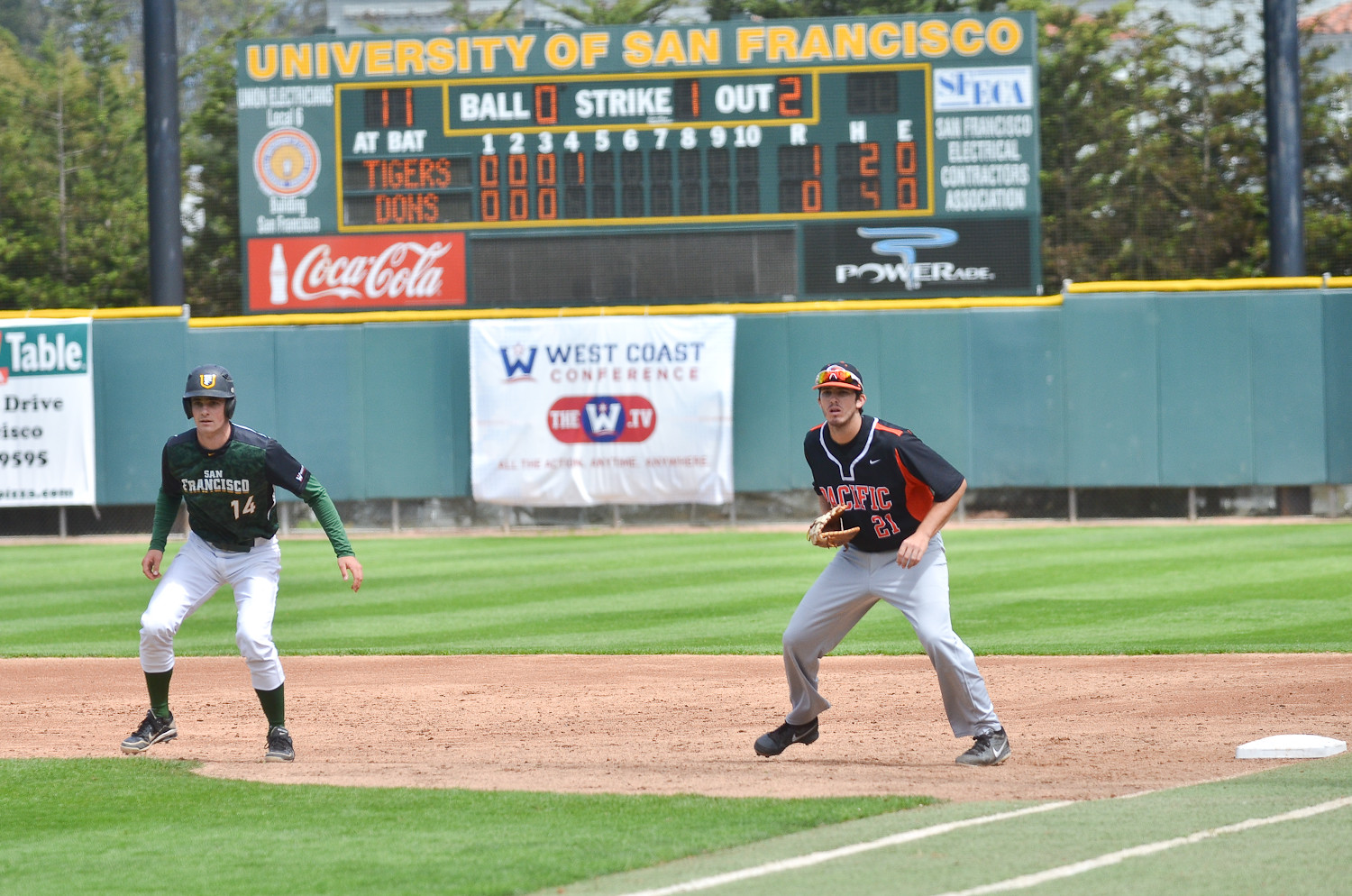The image captures a lively baseball game at a stadium, with the University of San Francisco prominently displayed in yellow text atop the green scoreboard. The scoreboard details the game between the Tigers and the Dons, showing the Tigers are leading with one run while the Dons have none. The current batter is number eleven, with the count at zero balls, one strike, and two outs. Advertisements for Coca-Cola and Powerade add a splash of color to the scoreboard, while additional ads for the West Coast Conference are visible in the background.

On the field, two players are central to the action. The first baseman, dressed in black and orange, is looking ahead, ready and focused. Nearby, a runner, clad in green, black, and white, is taking a lead, also intently focused on the game. The green outfield wall features several white signs along the right field side. Behind the vibrant scene of the field and players, a serene line of trees provides a natural backdrop, contrasting with the competitive energy of the game.